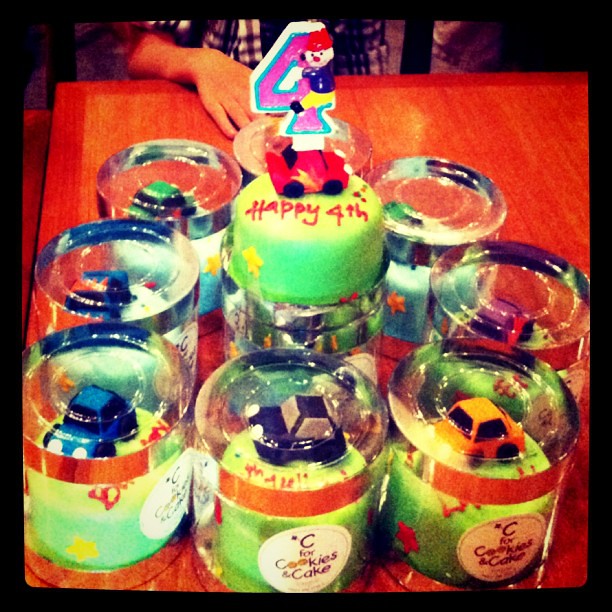The digital photo captures an indoor scene celebrating what appears to be a fourth birthday. Dominating the bottom center of the image is a large green cake decorated with the red-scripted message "Happy Fourth." The cake features a Lightning McQueen car from the movie "Cars" with a number four and a small cartoon character on top, symbolizing the birthday milestone. Surrounding the large cake are eight clear jars, each containing green frosted mini-cakes or cookies. These jars are labeled with white circular stickers that read "C for Cookies and Cake" in black font. Each mini-cake is adorned with colorful toy cars, including yellow, blue, and purple varieties. The scene is set on a reddish-orange wooden table, upon which a child with a light skin tone rests their right hand. The child, who is wearing a blue and white checkered shirt, stands in front of the table, completing this festive birthday tableau.